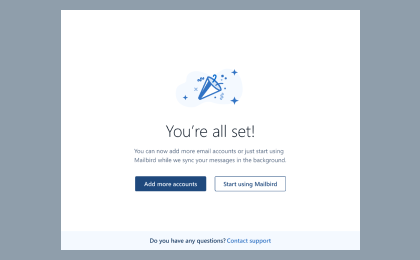The image depicts a confirmation screen for the Mailbird application. The background is a neutral gray, which helps to highlight a prominent white box in the center. Inside this white section, there is a celebratory party icon, indicating success. The text reads, "You're all set. You can now add more email accounts or just start using Mailbird while we sync your messages in the background." Below this message, there are two prominent buttons: a blue "Add More Accounts" button and a secondary "Start Using Mailbird" button. At the bottom of the white box, the text prompts, "Do you have any questions?" with a hyperlink to contact support. This screen signifies that Mailbird has been successfully set up and is ready for use, offering options to either add additional email accounts or begin using the application immediately. The overall layout is clean, straightforward, and functional, ensuring users can clearly understand that their setup process is complete.